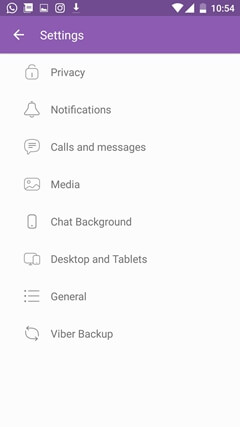This image is a detailed screenshot of a mobile phone's settings page. The image is rectangular in shape, resembling the aspect ratio of a phone screen, with no visible borders. The layout of the settings screen is divided into three main sections: a deep purple header, a lavender sub-header, and a light gray background that dominates the majority of the space.

At the very top, the deep purple header features several white icons. From left to right, these icons include a circle with a telephone, a square with an indistinct symbol, a bar chart, the standard settings gear, a download arrow, a clock displaying the time "10:54," a vertical battery icon indicating 40% charge, a right triangle, and a fully filled diamond-shaped Wi-Fi icon.

Below this header is a lighter purple, lavender-colored sub-header that is about three times the height of the deep purple header. This section contains a left-pointing arrow and the word "Settings" in white, aligned to the left side of the field.

The main body of the image consists of a light gray background that occupies approximately 80% of the total image area. This section features eight rows, each containing an icon and corresponding text, all in gray tones. The icons are slightly indented from the left edge, and the text is further indented.

1. **Privacy**: Represented by a lock icon.
2. **Notifications**: Displayed with a bell icon.
3. **Calls and messages**: Illustrated with a quote bubble icon, though only the "C" in calls is capitalized.
4. **Media**: Shown with an image icon resembling an outdoor landscape photograph.
5. **Chat Background**: Depicted with the outline of a mobile phone, both "C" and "B" are capitalized.
6. **Desktop and Tablets**: Identified with icons representing the screens of a desktop and a tablet, with both "D" and "T" capitalized, and the word "and" spelled out.
7. **General**: Indicated by an icon consisting of three stacked horizontal lines, each with a small square on the left.
8. **Viber Backup**: Marked by a continuous replay icon composed of two arrows forming an oval, with both "V" and "B" capitalized.

The bottom 20% of the image is an empty space, giving a clean end to the settings page.